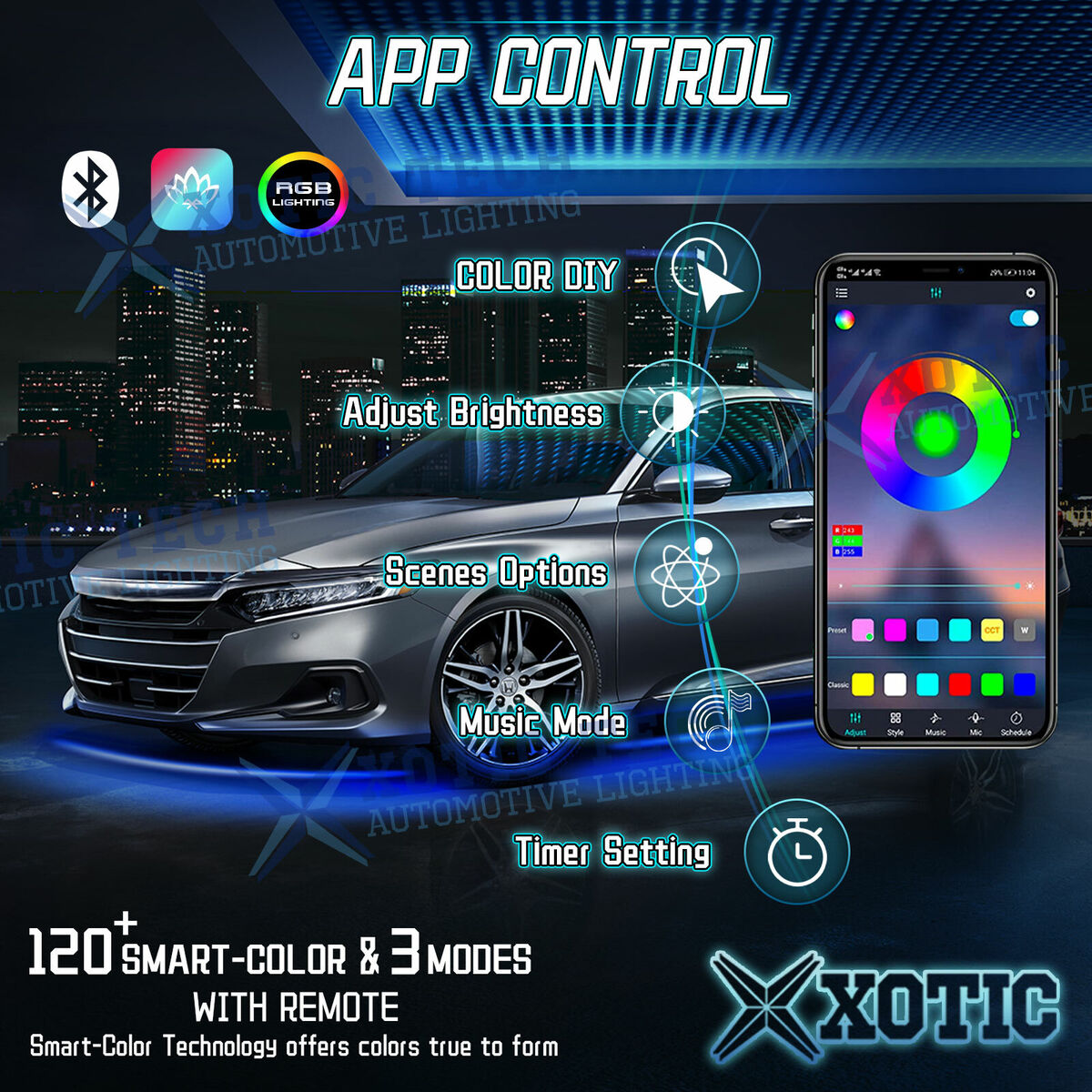The image is a detailed digital ad showcasing a car and an accompanying smartphone app. Prominently featured at the top is the white text "App Control" with a black outline and a blue glow. A silver Honda vehicle is displayed in the background. Below the main text, the ad highlights various features of the app, each represented by small icons. These features include "Color DIY," "Adjust Brightness," "Scene Options," "Music Mode," and "Timer Settings" — the timer symbol featuring a white outline of a car. In the top-left corner, alongside a Bluetooth symbol, there's an RGB lighting symbol displaying colors like purple, blue, green, yellow, and red. 

On the phone screen shown in the ad, there's a vivid color wheel, indicating that users can change the colors through the app. In the bottom-left corner, the text reads "120+ Smart Color and Three Modes with Remote. Smart Color Technology Offers Colors True to Form." In the bottom right, the brand logo "Xotic" is displayed, with a stylized "X" reminiscent of a compass. Overall, the ad effectively promotes the advanced lighting control features available for the car through the app, emphasizing ease of use and precise color customization.